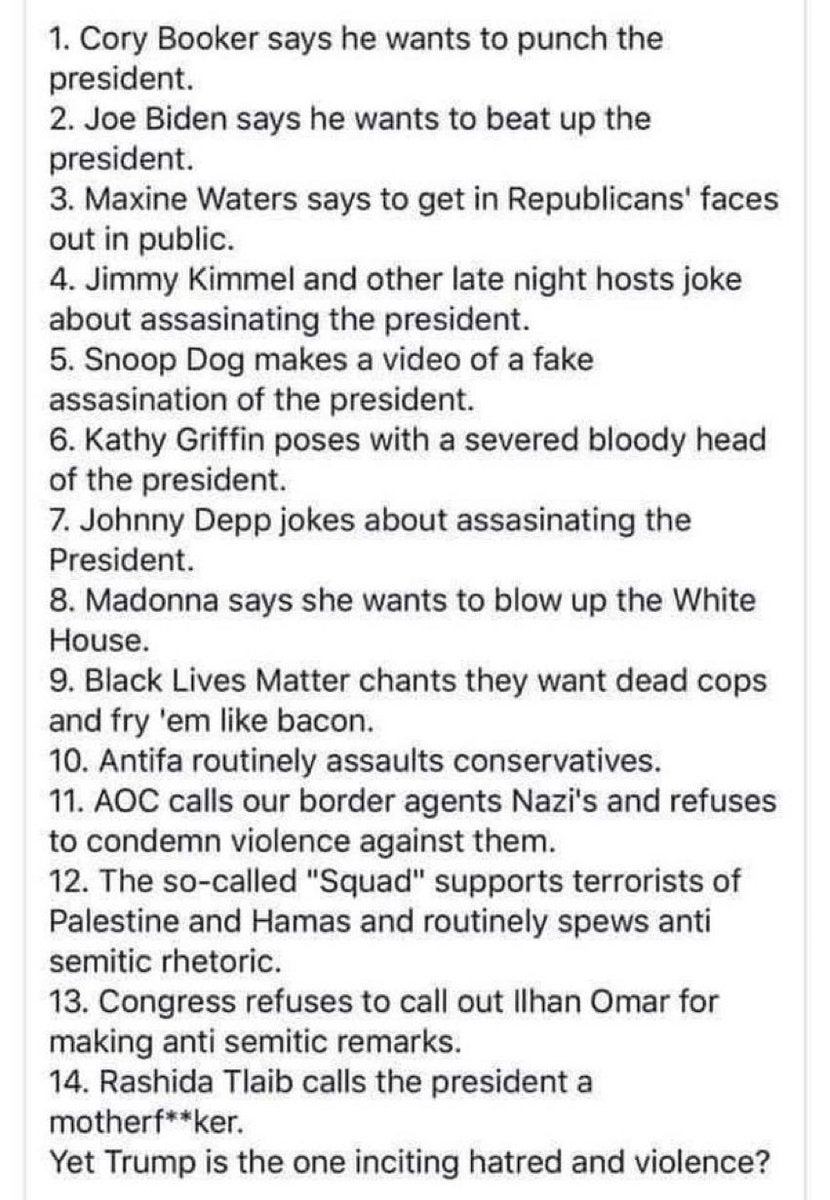A screenshot of a phone has been captured, revealing a stark white background with subtle light gray vertical lines on both the left and right sides. The central focus of the screenshot is a list numbered from 1 to 14, depicting various statements and actions attributed to different individuals, predominantly political figures and celebrities, that suggest or incite violence. The entries include:

1. Cory Baker expressing a desire to punch the president.
2. Joe Biden stating he wants to beat up the president.
3. Maxine Waters encouraging confrontational behavior towards Republicans in public.
4. Jimmy Kimmel and other late night hosts making jokes about assassinating the president.
5. Snoop Dogg creating a video depicting a fake assassination of the president.
6. Kathy Griffin posing with a faux severed, bloody head resembling the president.
7. Johnny Depp joking about the potential assassination of the president.
8. Madonna expressing thoughts about blowing up the White House.
9. Black Lives Matter chanting for dead cops and inciting violence.
10. Antifa routinely assaulting conservative individuals.
11. AOC likening border agents to Nazis and not condemning violence against them.
12. The so-called squad supporting Palestinian and Hamas-linked terrorists while frequently spewing anti-Semitic rhetoric.
13. Congress refusing to call out Ilhan Omar for making anti-Semitic remarks.
14. Rashida Tlaib labeling the president a "mother effer."

At the bottom of this list, logically separated yet emphasizing its point, is a statement suggesting that former President Trump is being accused of inciting hatred and violence, despite the aggressive actions and comments listed above. This entry does not carry a number, contrasting with the other items on the list that are sequentially numbered.